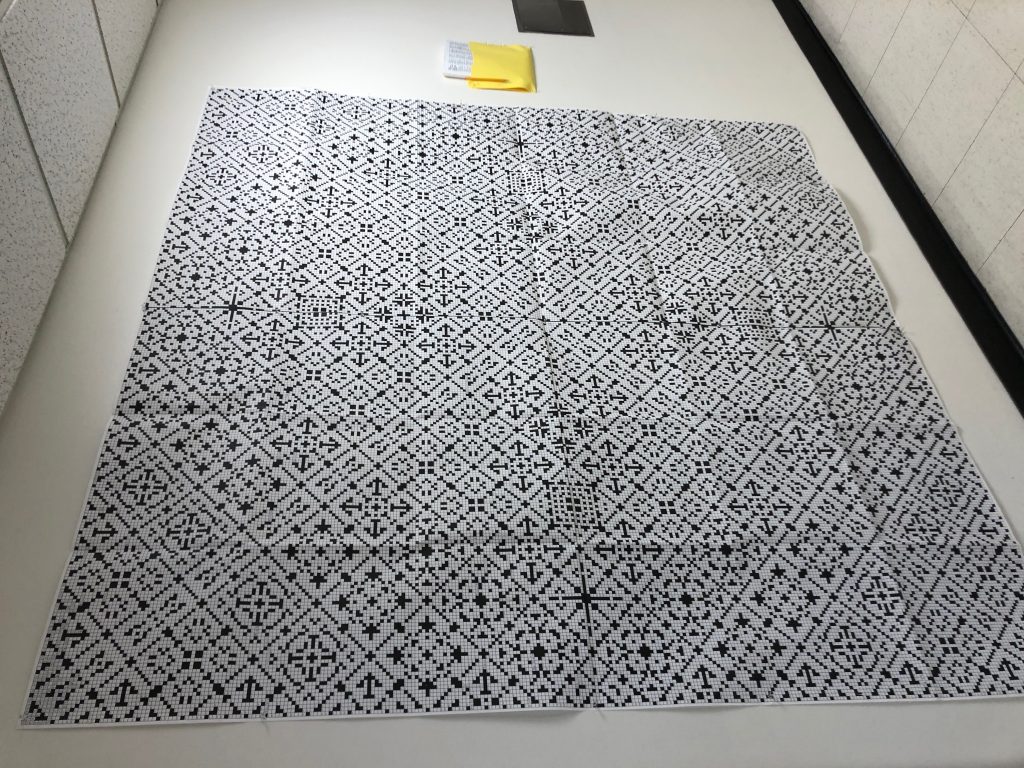This image depicts a small, white-tiled hallway or bathroom with tiled walls on both sides made of vertical, white, rectangular tiles. Near the bottom of the right wall, there's a horizontal black strip running along the baseboard. The main focus is a large black and white mat or quilt in the center, decorated with various intricate patterns, including crosshairs, arrows, stars, and squares, resembling a bandana design. Above the mat on the wall, there is a folded yellow rag or envelope with a white strip on its left end, positioned beneath a black square. The overall impression is one of minimalistic design with a striking central textile feature, creating a balanced contrast with the surrounding plain white tiles.